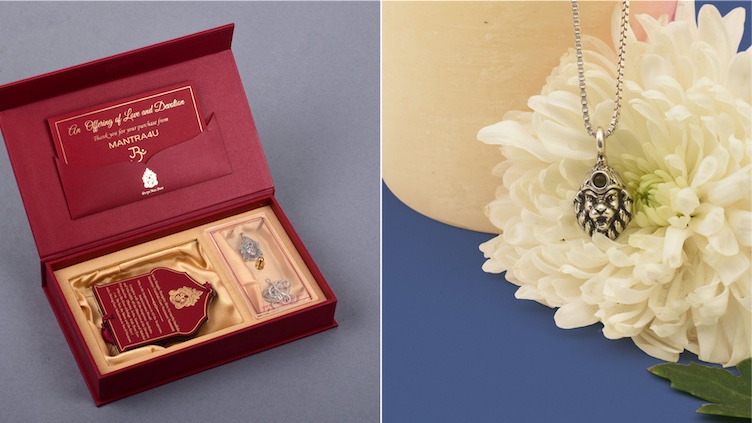This detailed photograph showcases two images separated by a thin white line. On the left, an open red gift box rests against a blue background, revealing its luxurious gold interior. Inside, there is a red business card with intricate, unreadable text, a red tag with script detailing the item's significance, and a medallion adorned with a lion's head logo. On the right side of the image, set against a rose gold background, is a person wearing a blue shirt, their neck adorned with an elegant silver pendant necklace. The pendant, designed to resemble a lion's head, features a black gem at its center and dangles from a silver chain. This scene is complemented by a large, detailed white chrysanthemum, verdant green leaves, and a hint of blue in the upper right corner. The image on the right symbolizes the complete gifting experience, encapsulating love and luxury.